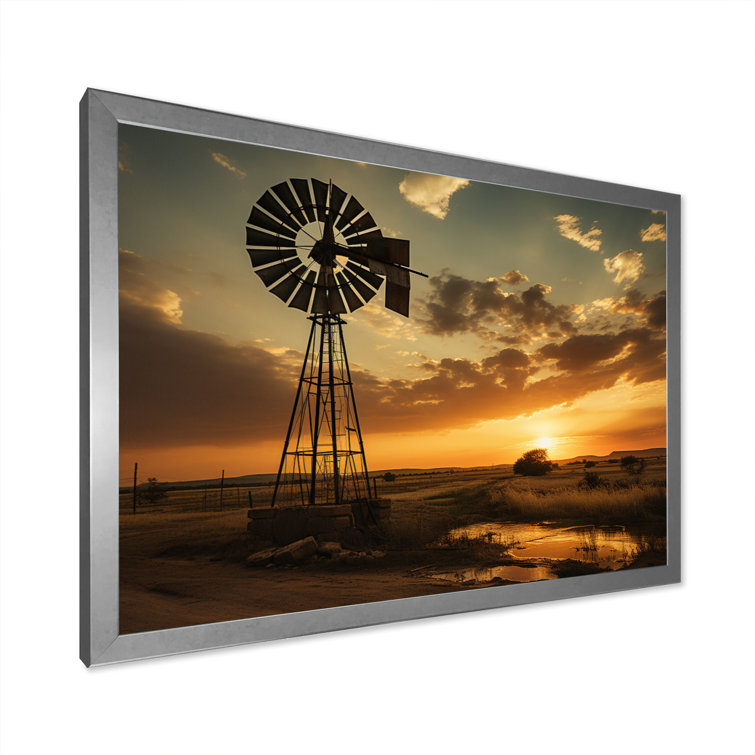The image depicts an art piece on a white wall, framed by a silver, metallic structure that could resemble a modern photo frame or a flat-screen television. The central photograph within this frame showcases a serene rural scene at sunset. The focal point is an older-style metal tower, reminiscent of a weather vane or rustic windmill, situated slightly to the left of the image. The sky behind it is a light blue, interspersed with gray clouds tinged by the orange and yellow hues of the setting sun, which is descending toward the right-hand side of the frame. Below this picturesque sky, a flat expanse of land stretches out, dotted with grass, weeds, and a few scattered fence posts. The land seems to be lit with a soft, orange glow from the sunset. Adding to the tranquility, there is a small puddle or pond reflecting the warm colors of the horizon, enhancing the peaceful ambiance of this rural landscape.